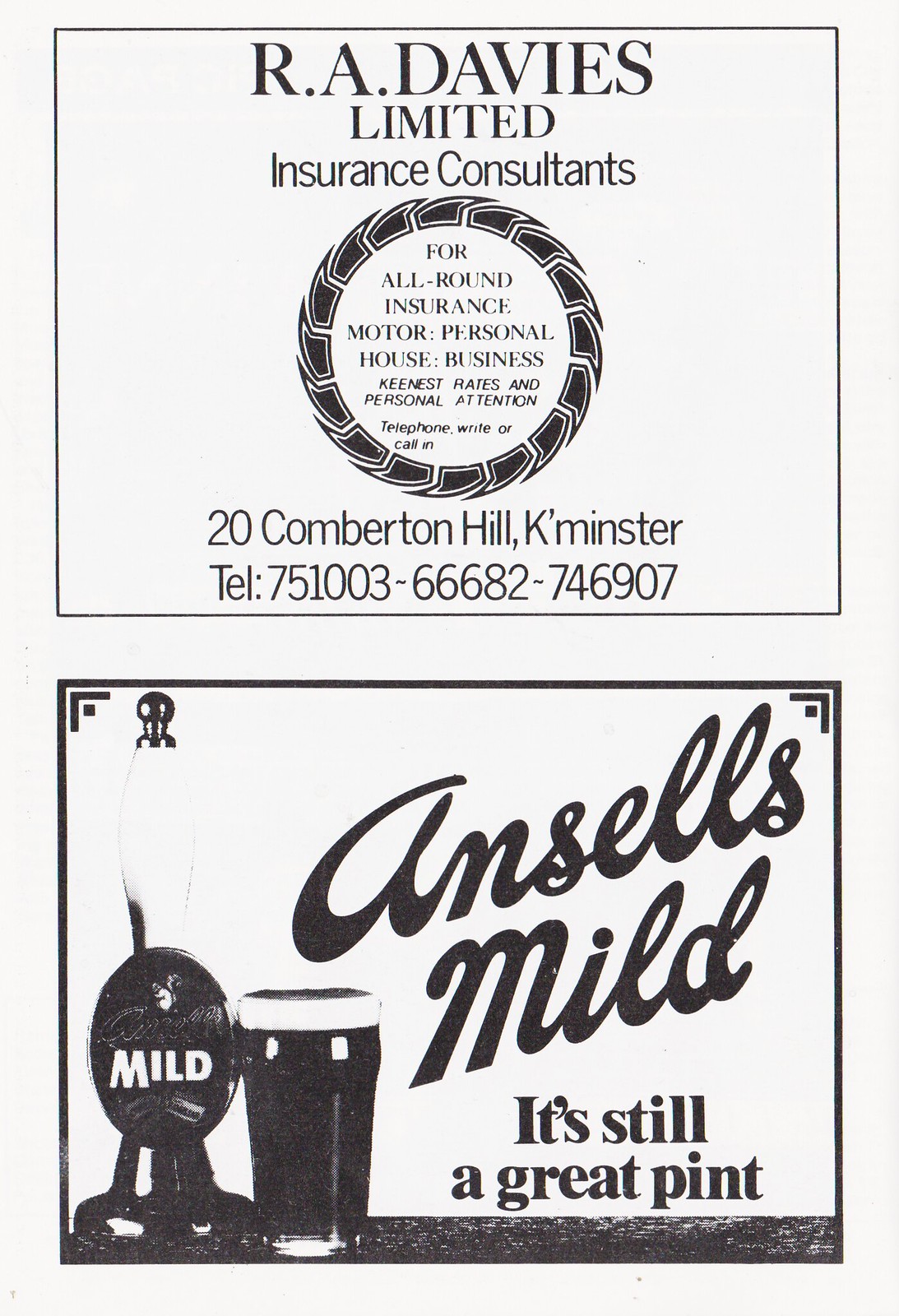This black and white magazine or program page, likely from several decades ago, features two vertically stacked advertisements. The top advert is for R.A. Davies Limited Insurance Consultants, prominently displaying the company's name in large, center-justified text. Enclosed within a circular design resembling a spiked or thorn wreath is detailed text promoting their comprehensive insurance services: motor, personal, house, business, boasting keenest rates and personal attention. Below this circular element are the company’s address and telephone number.

The bottom half of the page showcases a nostalgic advertisement for Ansel's Mild, boldly declaring "It's still a great pint." Accompanying this slogan is an image of a full beer mug, positioned to the left, with a beer tap bearing the drink's logo poised above it. The classic styling of both advertisements suggests the page dates back several decades, evoking a historical charm.